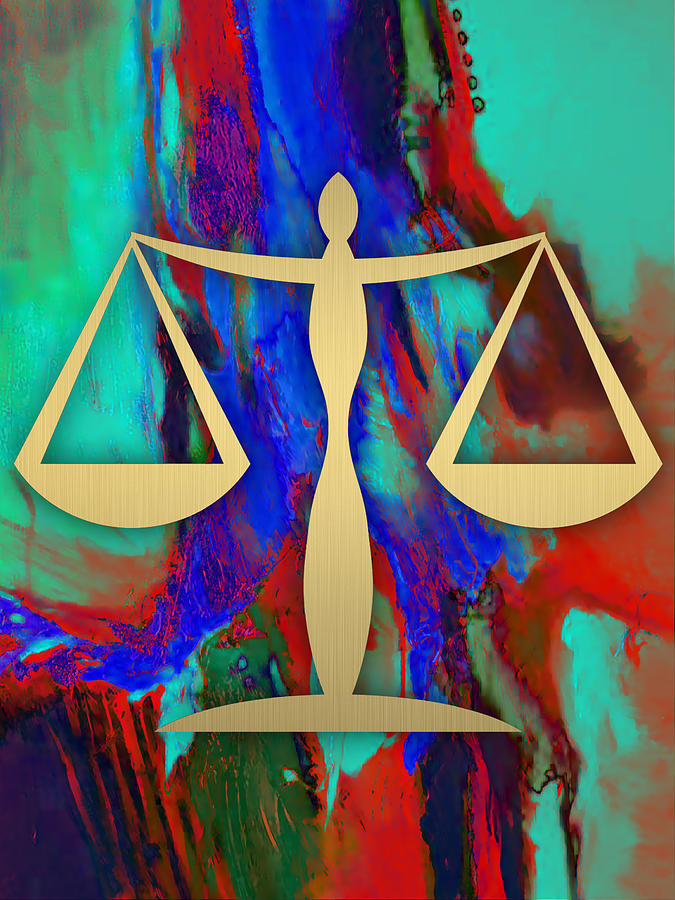This vibrant, abstract painting showcases a dynamic background featuring a myriad of bright colors, including prominent streaks and swirls of turquoise, red, blue, green, and a touch of black. Turquoise is most prominent, particularly visible at the top right, bottom right, and a long streak extending from the top left. The middle section features a slightly printed or stenciled gold scale, symbolizing balance or justice, with two arms outstretched holding baskets on each side. The gold scale stands in stark contrast to the colorful background, making it a striking focal point. The overall composition is a blend of vivid hues and abstract forms, giving it a unique and captivating appeal.